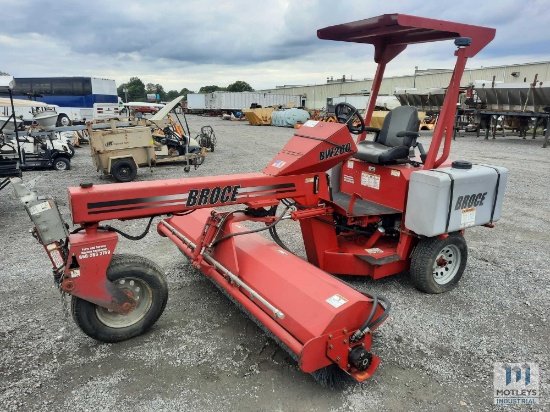This outdoor image captures a red piece of tractor equipment with a black seat, a black steering wheel, and a protective red canopy top above the seat. The equipment features a single front wheel and two smaller rear wheels, giving it a tricycle-like appearance. The prominently displayed text "BROCE" with lines extending outward is visible on the side of the machine. Beneath and between the front and rear wheels, a long red attachment spans perpendicularly. The vehicle is situated on a gravel parking lot, which appears gray and white, and various other older pieces of equipment, a large truck trailer, a bus, and a warehouse made of sheet metal populate the background. The sky is overcast with many clouds, adding to the gray ambiance. In the lower right-hand corner of the image, there's an icon with "Motley's Industrial" and three vertical blue stripes. The colors in the scene include blue, gray, white, red, orange, and tan.